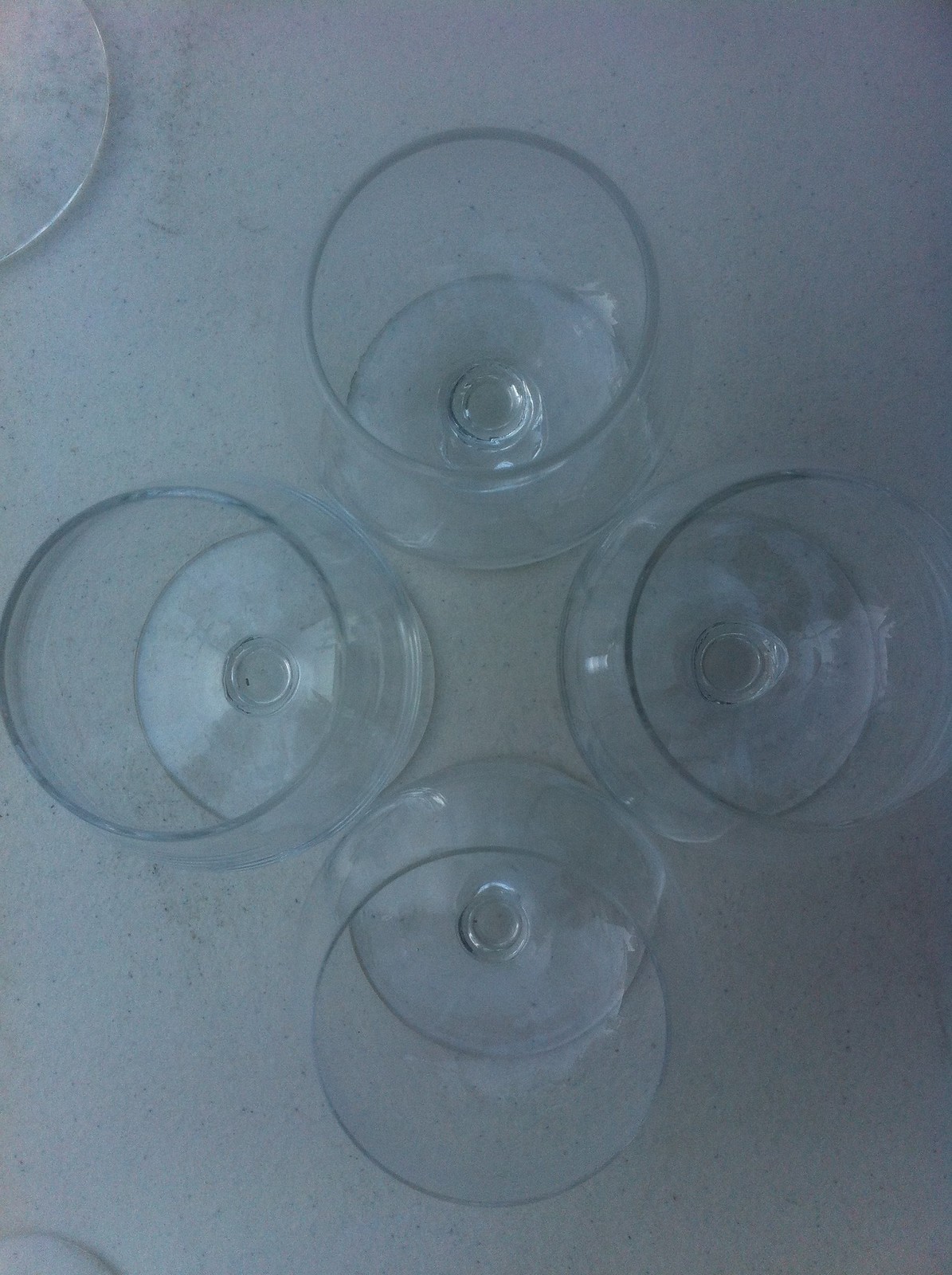This photograph captures an overhead view of four clear, round glasses arranged in a diamond pattern on a speckled off-white and gray surface, which could be a floor, table, or tablecloth. Each glass is translucent with reflective surfaces and exhibits depth at the brim. Some glasses appear slightly spotted or dirty, and it is difficult to determine if there is any liquid inside, though there might be a small amount of water. In the upper left-hand corner, there is the stem of another glass, partially cut off by the edge of the image, and in the lower left-hand corner, an indistinct circular object can be observed on the gritty surface.